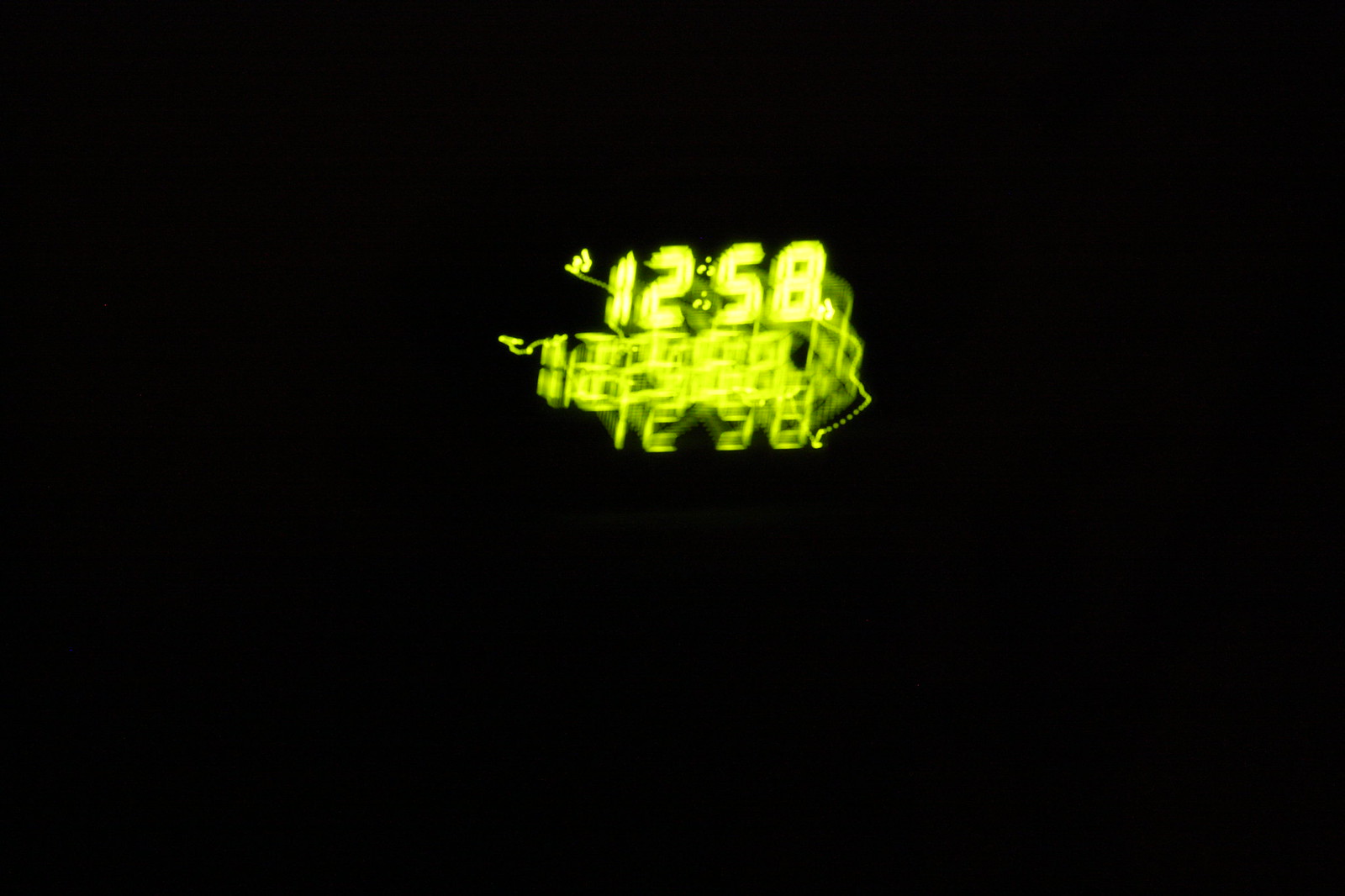The image predominantly features a pitch-black background with a central cluster of bright digital clock readings. The clock displays the time "12:58" in a neon green hue, which appears repeatedly in a layered, blurred effect, suggestive of either long exposure or multiple exposures. This creates a blended, mesh-like appearance of the numbers, with some swirls and streaks to the right. The numbers at the top center are more distinct, while those below become progressively more blurred, overlapping each other. Despite the dense layering of the digital readouts, the image maintains a minimalistic look with the black background, accentuating the central, chaotic cascade of illuminated time.